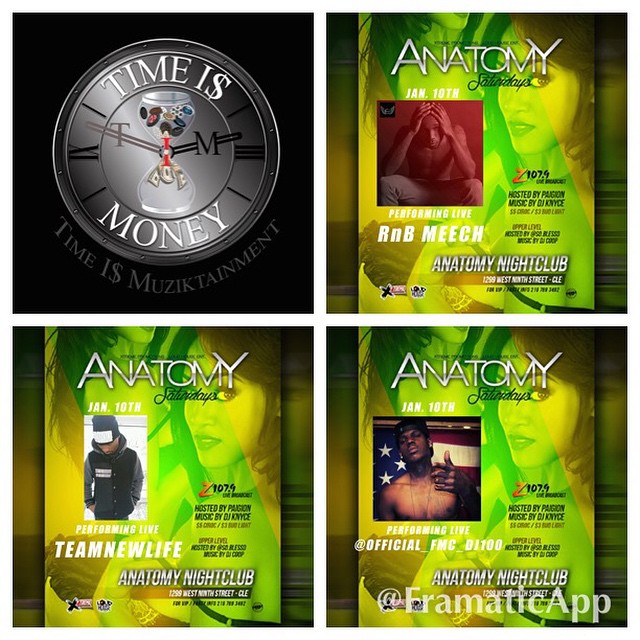The image is a four-panel design, with each panel serving a distinct purpose. The top left panel features an artistic watch face with the phrase "Time is Money" inscribed on it. The watch face is not functional but rather a design element, with an hourglass at the center displaying what appears to be buttons at the top and money falling at the bottom, symbolizing the flow from time to money. Below the watch face, the phrase "Time is Musictainment" is prominently displayed.

The other three panels resemble posters for events at Anatomy Nightclub, titled "Anatomy Saturdays." Each poster shares a common backdrop that includes an image of two women standing together, one glancing over her shoulder, viewed through a green and yellow filter. Each poster features a different male performer. The performers are labeled as R&B Meech, Team New Life, and @officialFMCD1100. Details about the event hosts, artists appearing, DJs, and supporting radio stations are displayed on the left side of the flyers. The predominant colors of the flyers are green, maintaining a cohesive theme across all event posters.